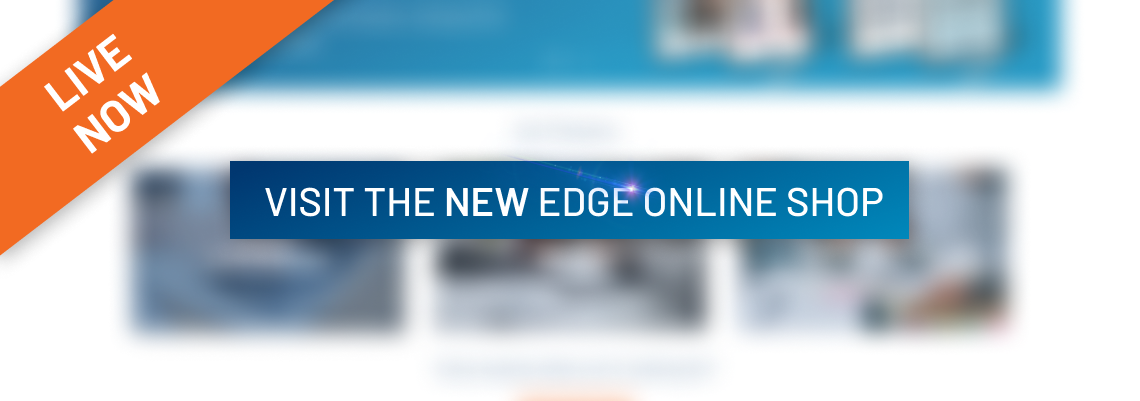A partially loaded webpage featuring a prominent "Live Now" notification and a promotional banner for the "New Edge Shop Online." This nascent online store remains ambiguous in purpose, potentially offering items ranging from medical supplies to workplace swag. The layout includes a blue banner spanning across the top, and an orange banner diagonally positioned in one corner. The background, slightly blurred, reveals a larger blue banner accompanied by several images of people engaged in various activities. Unfortunately, only the top quarter of the webpage has loaded, leaving the rest shrouded in mystery. However, it's clear that this is a newly launched e-commerce platform, inviting visitors to explore and make purchases.